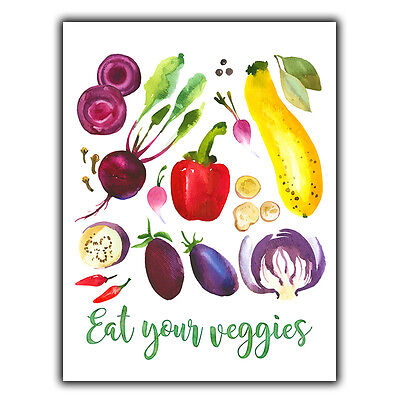This poster is a vibrant watercolor painting of various vegetables, designed to promote healthy eating. Set against a white background with a subtle black shadow border, the image features an array of colorful vegetables including peppers, eggplants, turnips, onions, cauliflower, potatoes, squash, beets, a red bell pepper, chili peppers, tomatoes, garlic, and a halved red cabbage. These vegetables are scattered artistically across the poster, with leafy greens accenting the upper right corner. The centerpiece message "Eat Your Veggies" is written in playful green cursive at the very bottom. This visually appealing poster serves as a simple yet striking reminder to incorporate more vegetables into your diet for better health.